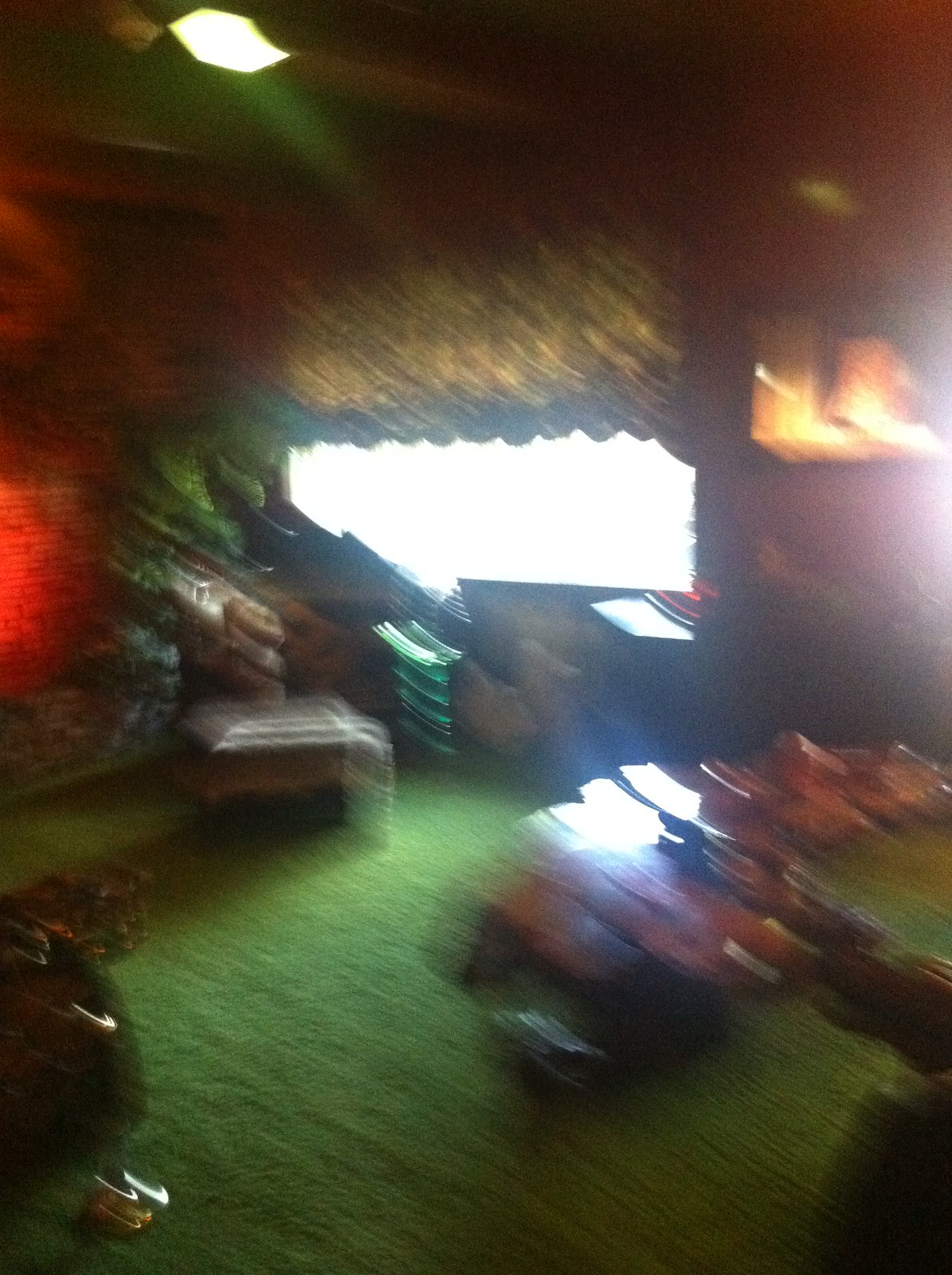The image depicts a room that evokes a nostalgic, old-fashioned atmosphere, perhaps reminiscent of a grandmother's house. The overall scene is very blurry, with a distinct directional blur that shifts elements down and to the side. The room features green carpet and orangey-red walls, contributing to the retro aesthetic. Amidst the blurred interior, a possible ottoman rests on the green floor, while a large, indistinct orange object occupies space nearby.

Central to the scene is a window, allowing a significant amount of light to flood in from the top left corner, possibly contributing to the image's haziness. Above the window hangs a curtain with a scalloped edge, appearing greenish, likely due to the light filtering through it. 

To the left, a mysterious red-glowing light suggests the presence of an exit sign or similar light source, with a green blur adjacent to it that could be an indoor plant. On the right side of the image, another orange blurred light adds to the room's hazy and indistinct look. This combination of elements and the peculiar blurring effect give the photograph a unique and slightly surreal quality.